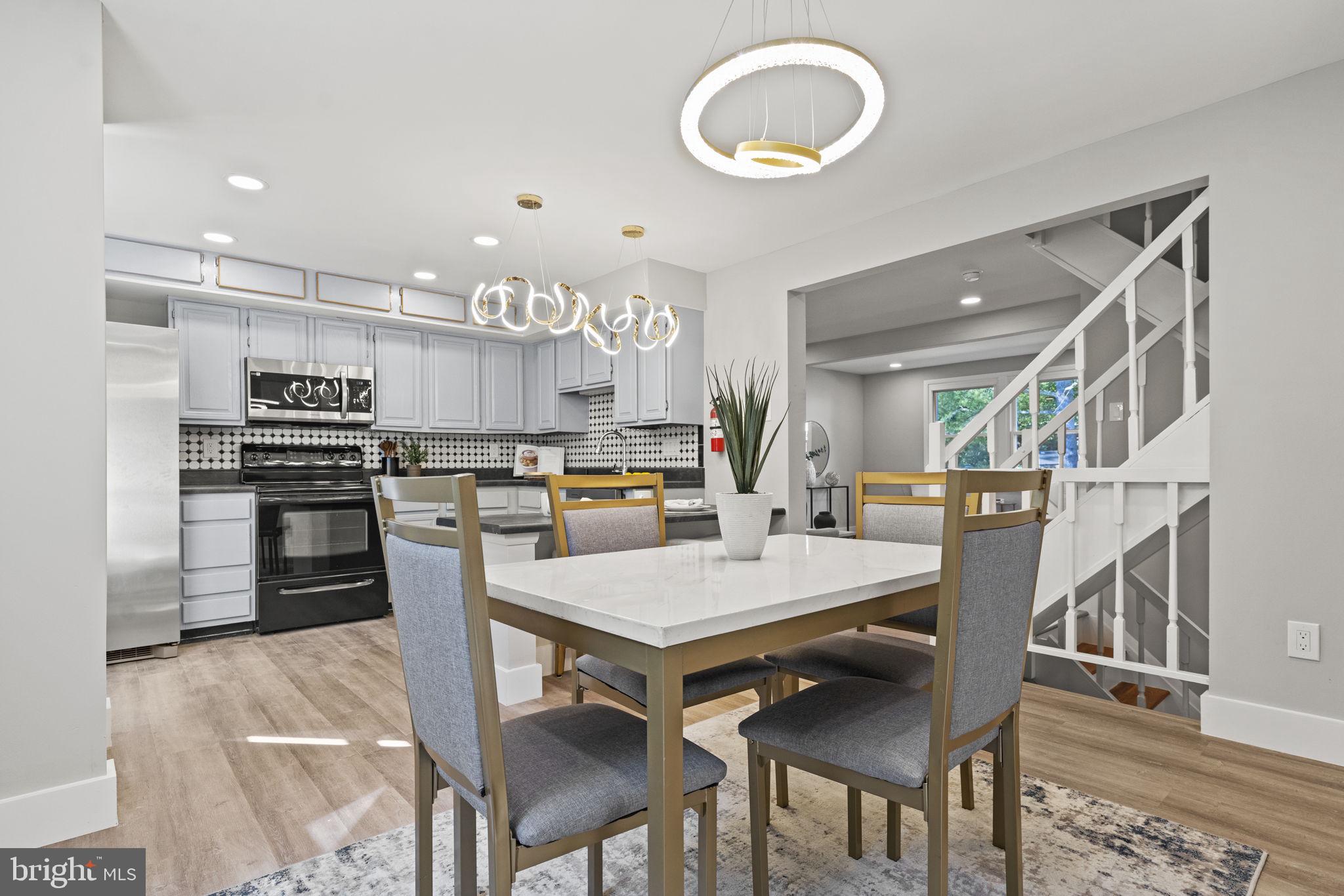The image showcases a meticulously designed open-concept dining room and kitchen area in a modern house, likely part of a real estate listing based on the “Bright, MLS” logo in the bottom left corner. The space is bathed in neutral tones, featuring light gray walls and white ceilings complemented by white crown molding and baseboards. A seamless transition of light-colored brown hardwood floors unites the two areas.

In the dining area, a chic table with a glossy white top, possibly made of quartz or marble, stands on gold-colored metal legs. Matching chairs with gold frames and heather gray fabric cushions are neatly arranged around the table, which sits on a multicolored rug with flecks of yellow, black, and white. A white flower pot with a green plant adds a touch of nature to the table’s centerpiece. Overhead, a modern circular light fixture with an inner ring hangs by wires, illuminating the table.

The adjacent kitchen features a mix of light and dark tones, with gray and white cabinets, a black stove, a stainless steel microwave, and a stainless steel refrigerator. The backsplash displays a black-and-white square pattern, adding texture to the space. An ornate, ribbon-like light fixture hangs over the kitchen island, adding further sophistication. Notably, a red fire extinguisher is mounted on the wall, ensuring practical safety features.

Behind the dining room, a white staircase with wooden treads leads upward, continuing the home's harmonious blend of materials and colors. In the distance, two windows bring natural light into the space, accentuating the room's airy feel. Recessed lighting throughout enhances the room’s contemporary ambiance, making it both stylish and functional.